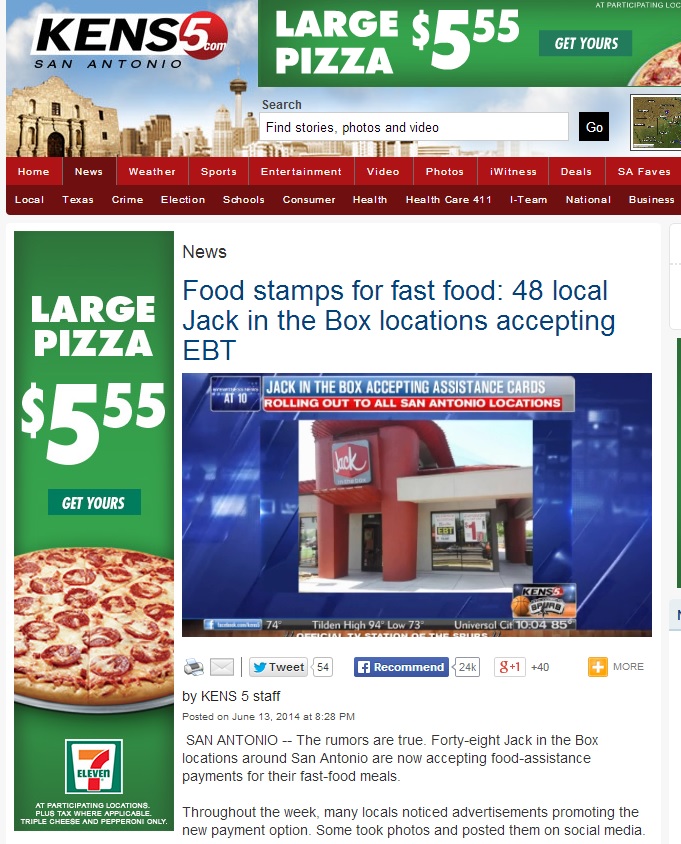This screenshot showcases a news article from KENS5.com, a San Antonio, Texas-based news broadcaster. The website design features a white background with a maroon and red navigation bar. Dominating the top of the page is a photograph of the iconic Alamo. In the top-right corner, there is a large green advertisement for pizza. Additionally, a vertical column along the left-hand side of the page displays another advertisement for the same pizza from 7-Eleven, prominently featuring a large pepperoni pizza image, priced at $5.55, and the 7-Eleven logo at the bottom.

The news article itself addresses a significant local update: 48 Jack in the Box locations around San Antonio are now accepting EBT (Electronic Benefit Transfer) payments for fast food purchases. Authored by the KENS5 staff, the article begins with the statement, "The rumors are true, 48 Jack in the Box locations around San Antonio are now accepting food assistance payments for their fast food meals." The article provides essential information on a change that will impact food assistance recipients in the area.